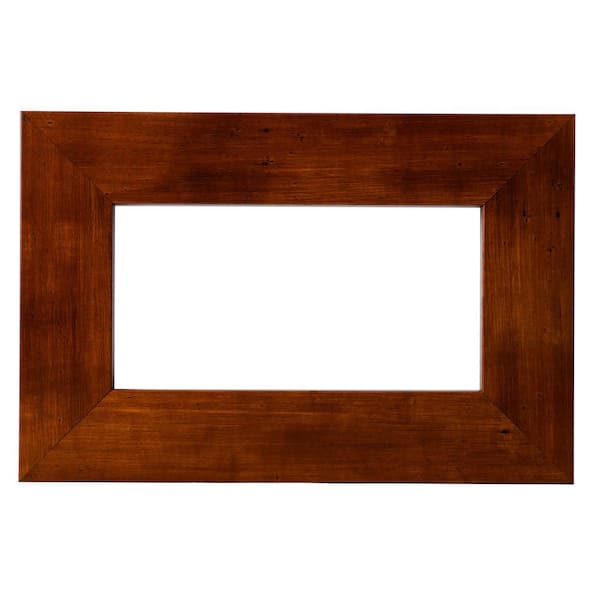The image depicts a beautifully polished and intricately detailed wooden frame, situated against a pristine white background. The frame is rectangular, showcasing a thick brownish-red wooden structure with a noticeable wood grain texture that adds to its charm. It has a significant width, almost half the height of its opening, creating a substantial and bold appearance. The inside of the frame is entirely empty, revealing a stark white void. The frame features sharp right-angle corners, each joined together with diagonal lines from the outer to the inner edges, contributing to its symmetrical and well-crafted look. Notably, the top and right sides exhibit a darker polish, while the bottom left corner has a subtle glow, hinting at the play of professional lighting and possibly a hint of gold tone shining through. This elegant wooden frame, with its reddish cherry wood hue and minor black spots along the grain, stands out as a testament to fine craftsmanship and attention to detail.